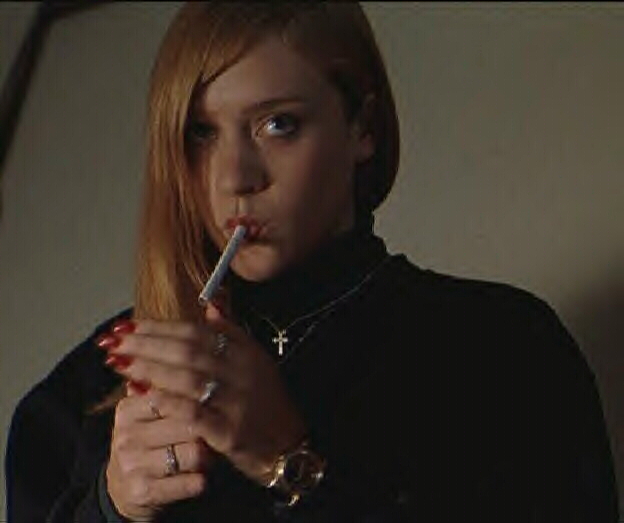The image captures a young woman with light skin and long, red hair that is parted and mostly falling over her right eye, while the left side is pulled back, exposing more of her face. She appears to be in the process of lighting a white cigarette that hangs from her mouth, using both hands to shield the flame; her nails are painted red, and she's adorned with several rings and a gold-faced, chunky watch. She wears a black jacket or possibly a sweater that comes up to her neck, and a silver necklace with a small gold crucifix hangs around her neck. Her expression is stern and somewhat unimpressed, looking slightly up towards the right. The background is an off-white or tan wall, though it's slightly dark and blurry, adding to the ambiance that may suggest a still frame from a movie due to the specific lighting effects in the image.